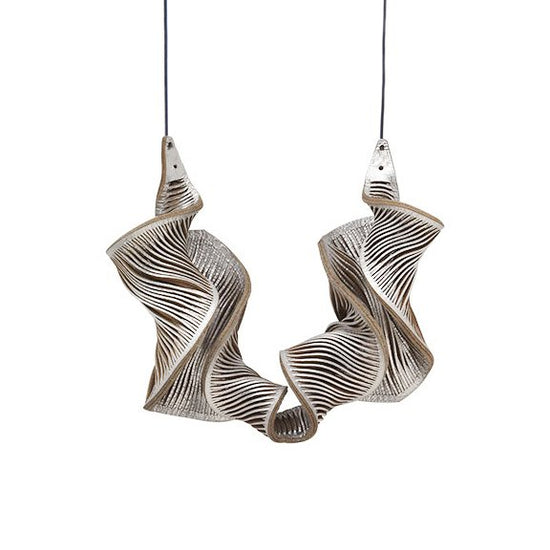The image features a hanging decoration suspended from the ceiling by two black strings. The main body of the decoration is a twisty, metallic-looking object with the rough shape of a U. Crafted from a material that mimics metal—likely painted cardboard or cloth—it exhibits bright, shiny silver surfaces that twist and curve elegantly, reminiscent of a ribbon. The bottom portion appears densely coiled, while the sides unfurl to the right and left, creating larger sections. Each larger section has interconnected lines that form the outer structure. At the top of these sections, there are small, white triangular pieces with buttons or lights, adding to the intricate design. These triangles have cords or extensions that protrude straight up from their tips. The overall aesthetic suggests a sophisticated, almost electronic appearance, with the entire object set against a stark white background, emphasizing its metallic gleam and detailed construction.